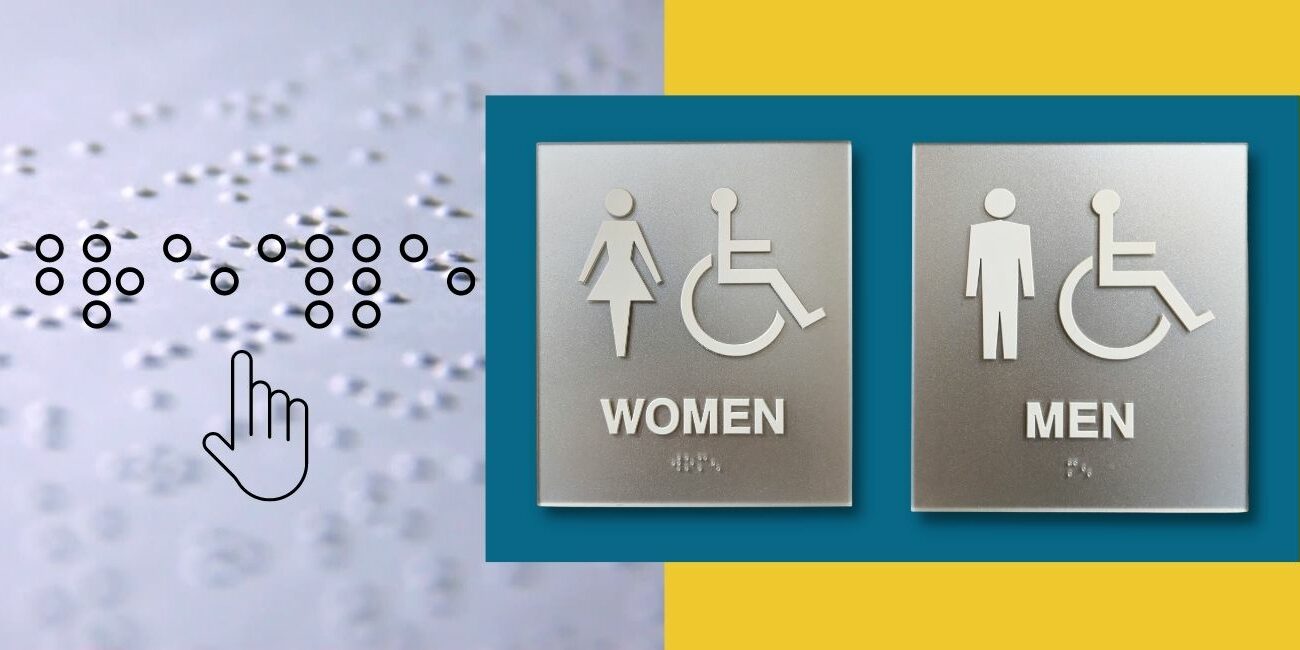The image displays two Braille-encoded restroom signs against a divided background. The left half of the background is a white square featuring raised white Braille dots, interspersed with black-clear dots forming readable Braille characters. Below the Braille, there's a black and white illustration of an upward-pointing hand. The right half showcases a bright yellow square overlaid with a turquoise rectangle extending slightly into the left half. This rectangle contains silver restroom signs for both men and women. The women's sign includes a stick figure in a skirt and a symbol for wheelchair accessibility, labeled "Women" with corresponding Braille underneath. Similarly, the men's sign features a stick figure in pants and a wheelchair symbol, labeled "Men" with its respective Braille below.